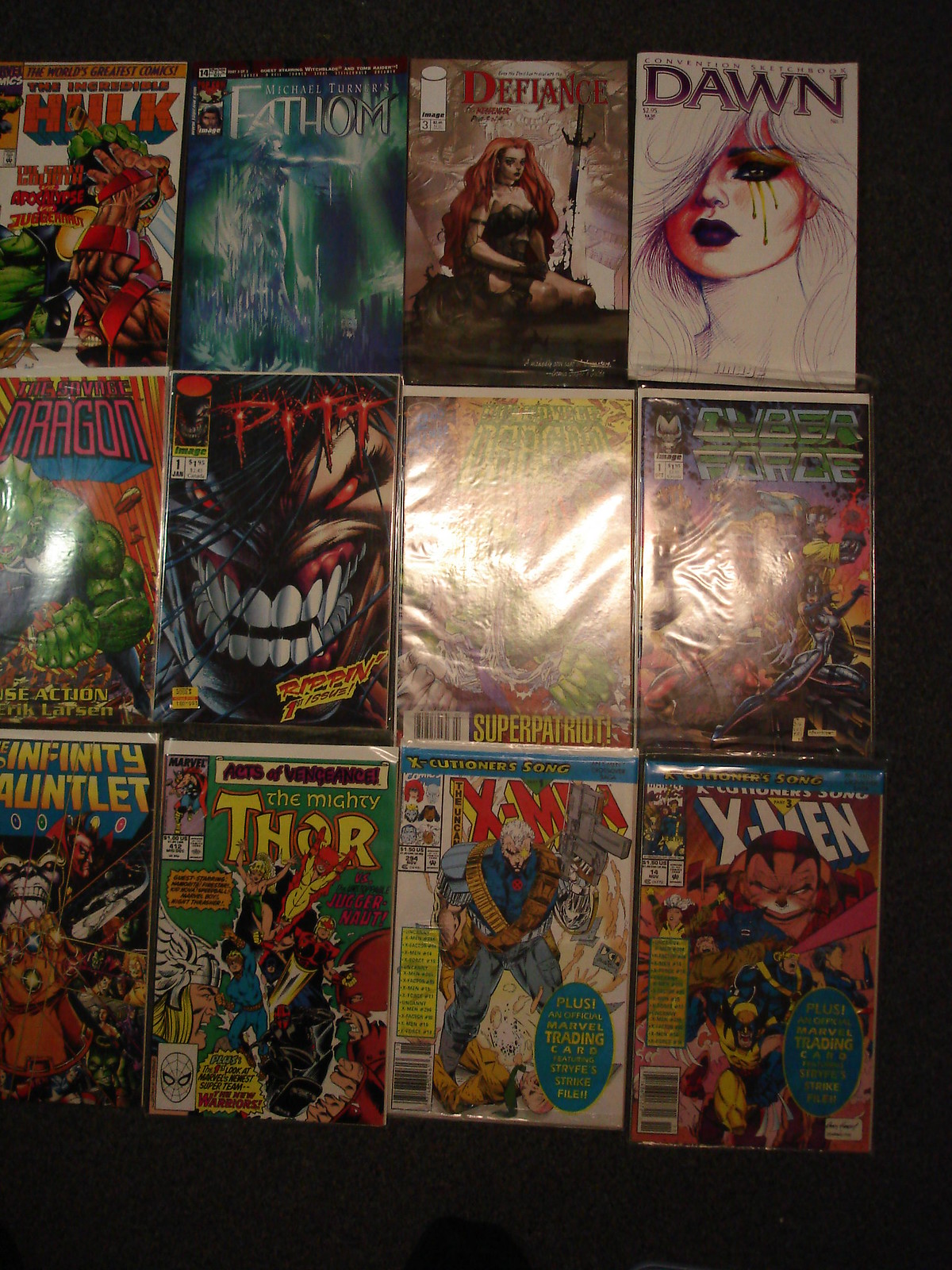The image displays a collection of 12 comic books arranged in three rows of four columns against a black background, which obscures the surface they are laid on. Each comic book appears to be encased in protective plastic, causing some glare. From left to right, the top row features "The Incredible Hulk," "Fathom," "Defiance," and "Dawn." The second row includes "The Savage Dragon," "Pit," another comic with a glare-covered title potentially identified as "The Savage Dragon" as well, and "Cyber Force." The bottom row presents "Infinity Gauntlet," "The Mighty Thor," and two "X-Men" comics.